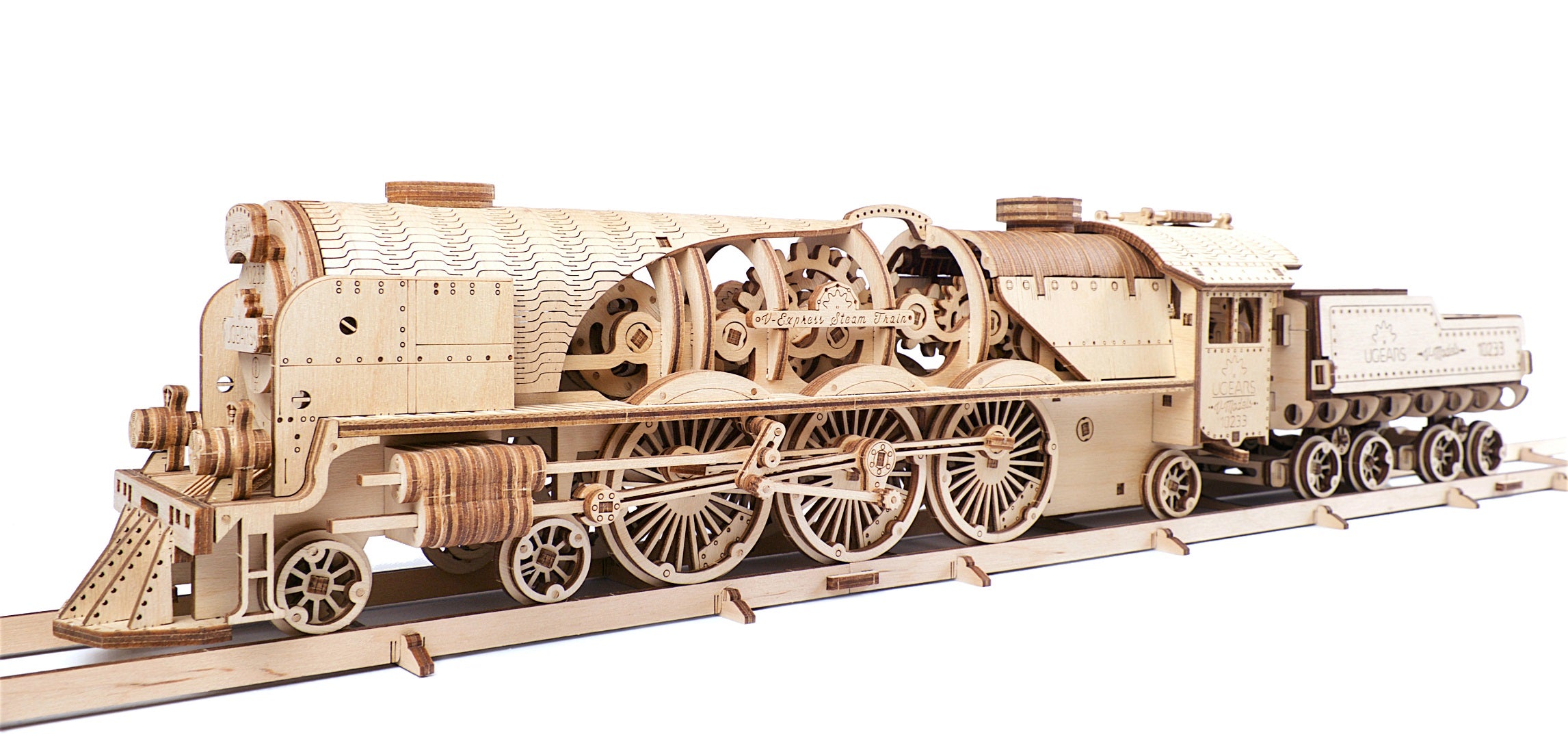The image showcases a meticulously crafted wooden model train set, highlighted against a pristine white background. The model, placed on a white table, features a wooden track stretching from the back right to the front left of the image. The train, constructed from light-colored wood and comprising hundreds of finely detailed pieces, includes a locomotive with a coal car attached. The locomotive, three to four inches wide and two inches high, reveals its intricate inner mechanics, with visible large gears and interconnected wheels. The train faces left and features three large wheels at the front, two small wheels behind, and a cow pusher. The train's body is partially open to display the gears that drive it. The engineer’s pilot house, located at the back of the locomotive, is white with two windows, leading to the attached coal car. The track, tan and off-white, is supported by six visible crosspieces, and the locomotive is adorned with dual smokestacks and black geometric patterns on its white upper front. The craftsmanship and detail suggest this train could be featured on a collector's site or for sale on a specialty platform like Etsy.